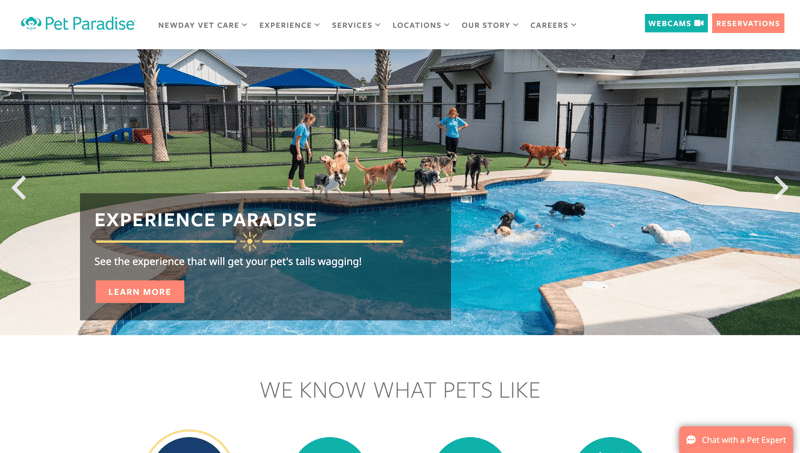The image is a screen capture from a web page displayed on a desktop computer screen, showcasing the "Pets Paradise" website. At the top left corner, the site name "Pets Paradise" is prominently written in green. To the right of the site name, a navigation bar features various web links labeled: "New Vet Care," "New Day Vet Care," "Experience," "Services," "Locations," "Our Stories," and "Careers." Adjacent to these links, there are two distinct buttons – a green "Webcam" button and an orange "Reservations" button.

Dominating the main section of the web page is a large image depicting a vibrant scene at Pets Paradise. The image features a kidney-shaped swimming pool filled with clear blue water. Several dogs are either playing joyfully in the water or standing by the poolside, some engaging with a ball. Behind the pool area, a lush green lawn extends, framed by a row of charming bungalows with white and gray walls. Adding a human element to the scene, two women, dressed in blue t-shirts and dark-colored pants, stand beside the dogs, overseeing the playful activity. The overall composition exudes a sense of fun, care, and relaxation in an idyllic pet-friendly environment.